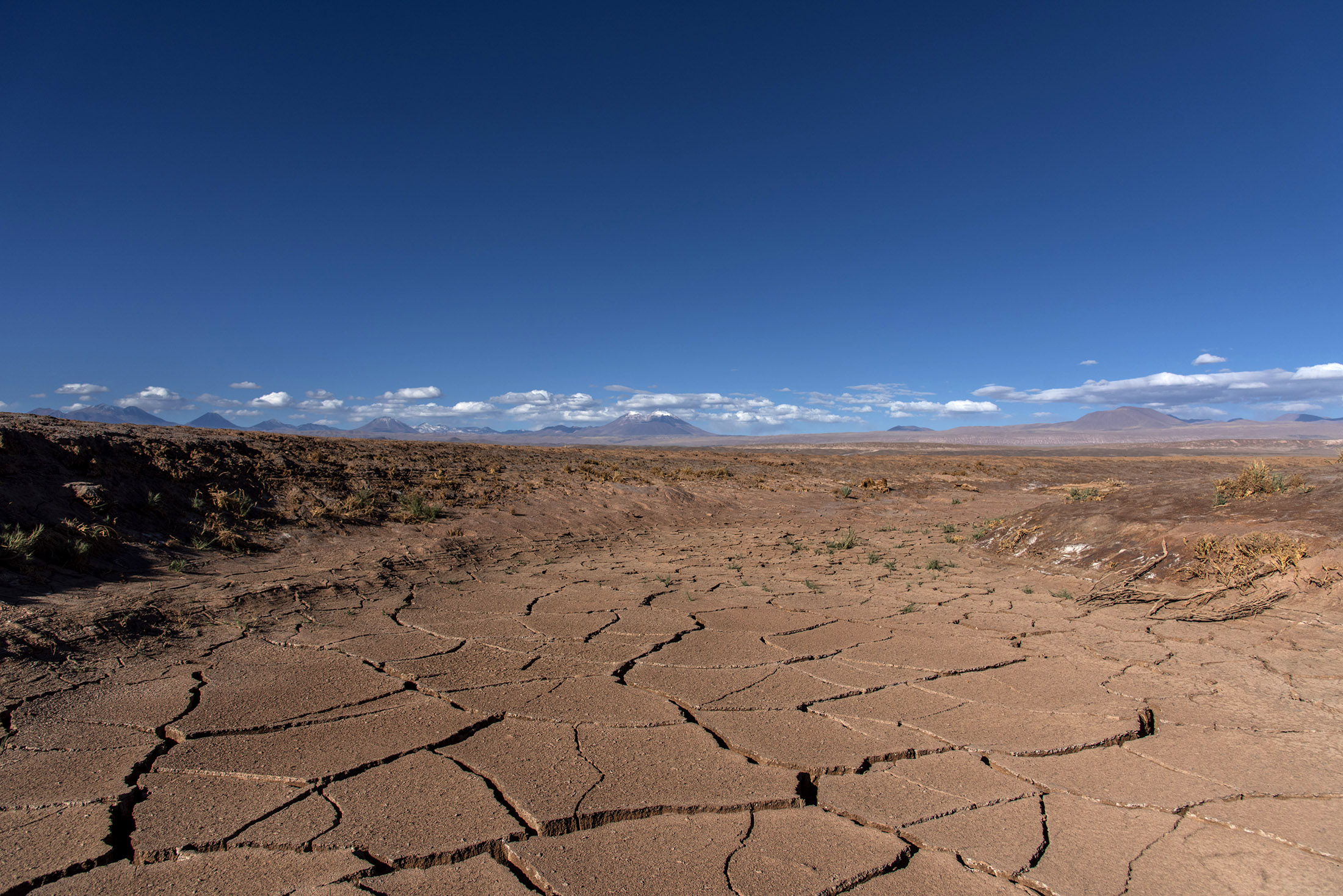This photograph captures a vast desert landscape under a clear blue sky with occasional white clouds touching the mountain range in the far background. The foreground prominently features a dry river basin or lake floor covered in large, cracked slabs of what appears to be fractured rock, indicating a recently dried-up body of water. The ground, predominantly light brown, extends far into the distance, emphasizing the desolation of the area. On the left-hand side, a slight hill with a dark brown, almost black tint is visible, sparsely adorned with patches of green vegetation. While scattered, dried-out grass persists on the right-hand side. The scene is devoid of people, enhancing the sense of solitude in this expansive, parched environment.